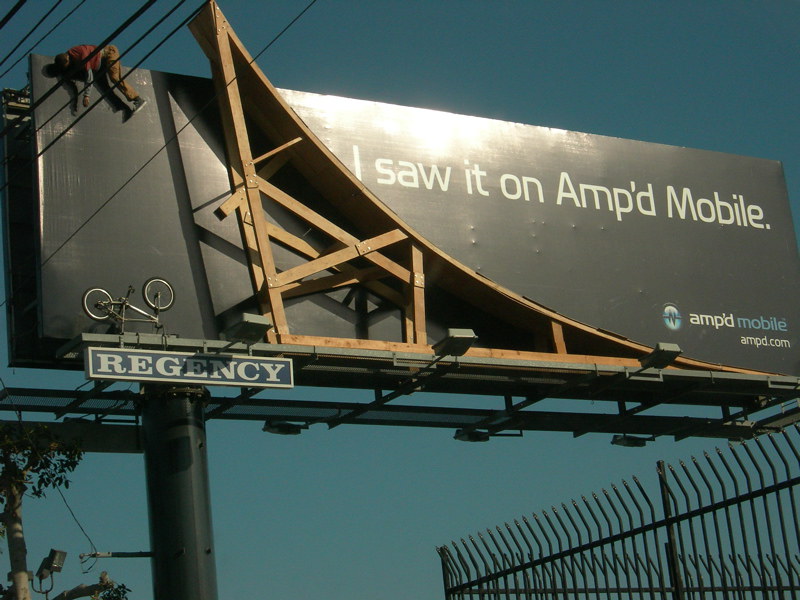This photograph features a billboard advertisement for Ampt Mobile. The billboard itself is primarily black and occupies the center of the image. On the left side of the billboard, there is a striking installation: a person dressed in red clothing and dark brown pants is slumped over the edge. Below them, an overturned bicycle can be seen, giving the impression of a dramatic accident.

The design of the billboard includes an impressive ramp structure, starting from the left and extending upward. This ramp suggests that the person was riding their bicycle along it, likely while distracted by their mobile phone, and ended up in their precarious position on the billboard.

The background showcases a vibrant blue sky, adding a sense of depth to the scene. There are no clouds to obscure the clear, sunny day. In the foreground, a sleek, black steel fence runs along the bottom edge of the image, adding another layer of context to this eye-catching advertisement.